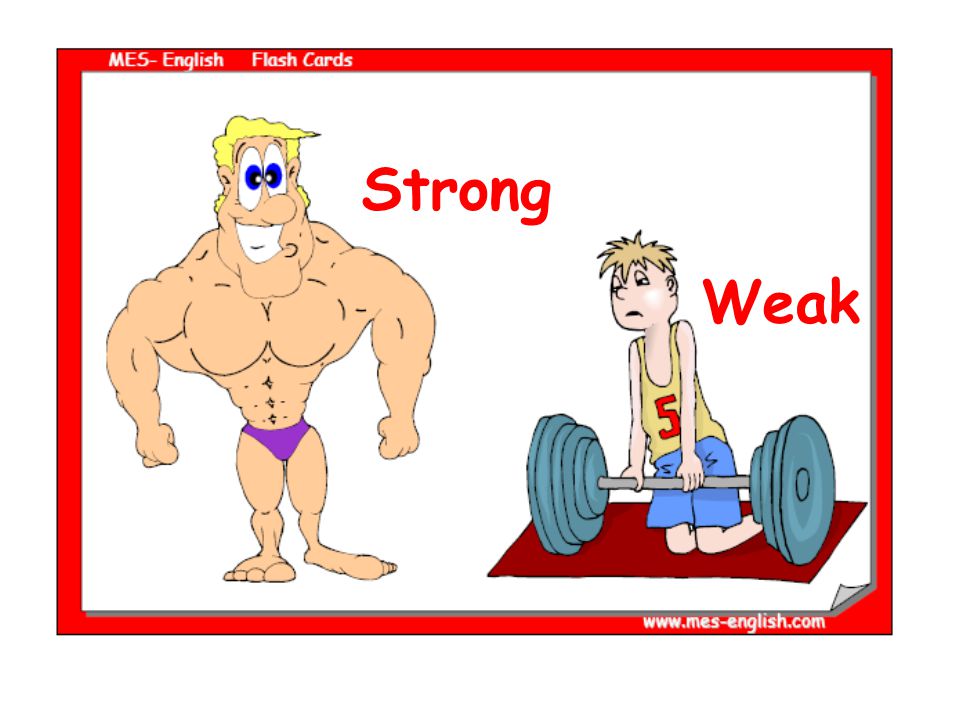This horizontal rectangular image, resembling more of a poster but referred to as a flash card, features a bright red border with white text. In the top left corner of the border, it reads "MES-English flash cards," and in the bottom right, "www.mes-english.com." The center of the image has a stark white background.

On the left side of the image is a cartoon figure of an overly muscular man with exaggerated features: short, curly blonde hair, big blue eyes, and a wide, goofy grin. He sports a small pair of purple Speedo swim trunks and flexes his bulging muscles. Next to his head, the word "strong" is displayed in bold red letters.

On the right side stands a much smaller, scrawny figure. This young boy has spiky light brown hair and wears a yellow tank top with a red number 5 on it, paired with blue shorts. He kneels on a red mat, struggling to lift a heavy barbell with teal weights. Beside him, the word "weak" is written in red text. The bottom right corner of the image appears slightly folded up.